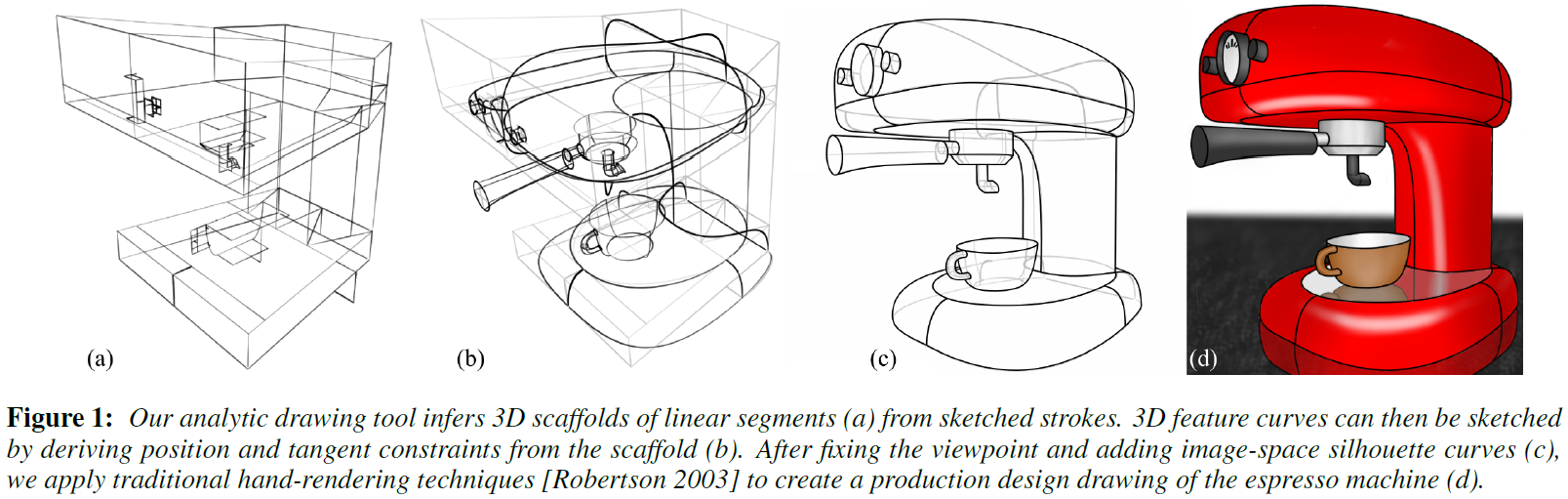The image presents a detailed step-by-step guide on creating a 3D model of a red espresso machine, illustrated through four progressive drawings labeled A to D. The top section of the image displays these sequential drawings on a white background: 

- **Drawing A** features the initial sketch of the coffee machine with straight black lines that form the basic structure.
- **Drawing B** introduces some curved lines, refining the sketch without losing the linear framework.
- **Drawing C** further enhances the model by incorporating more curves and reducing the emphasis on straight lines, shaping the design further.
- **Drawing D** is a colorful, final rendering of the espresso machine in red, complete with a black handle and a brown coffee cup placed underneath it. The machine and cup rest on a black surface.

The bottom section of the image contains descriptive text in black, explaining the drawing process. It reads as follows: "Figure 1. Our analytic drawing tool infers 3D scaffolds of linear segments A from sketched strokes. 3D featured curves can then be sketched by deriving position and tangent constraints from the scaffold B. After fixing the viewpoint and adding image space to the curved C, we applied traditional hand rendering techniques, Robertson 2003, to create a production design drawing of the espresso machine D." The image and text collaboration clearly illustrates the evolution from a simple line sketch to a detailed, colored design of the espresso machine, attributed to Robertson in 2003.